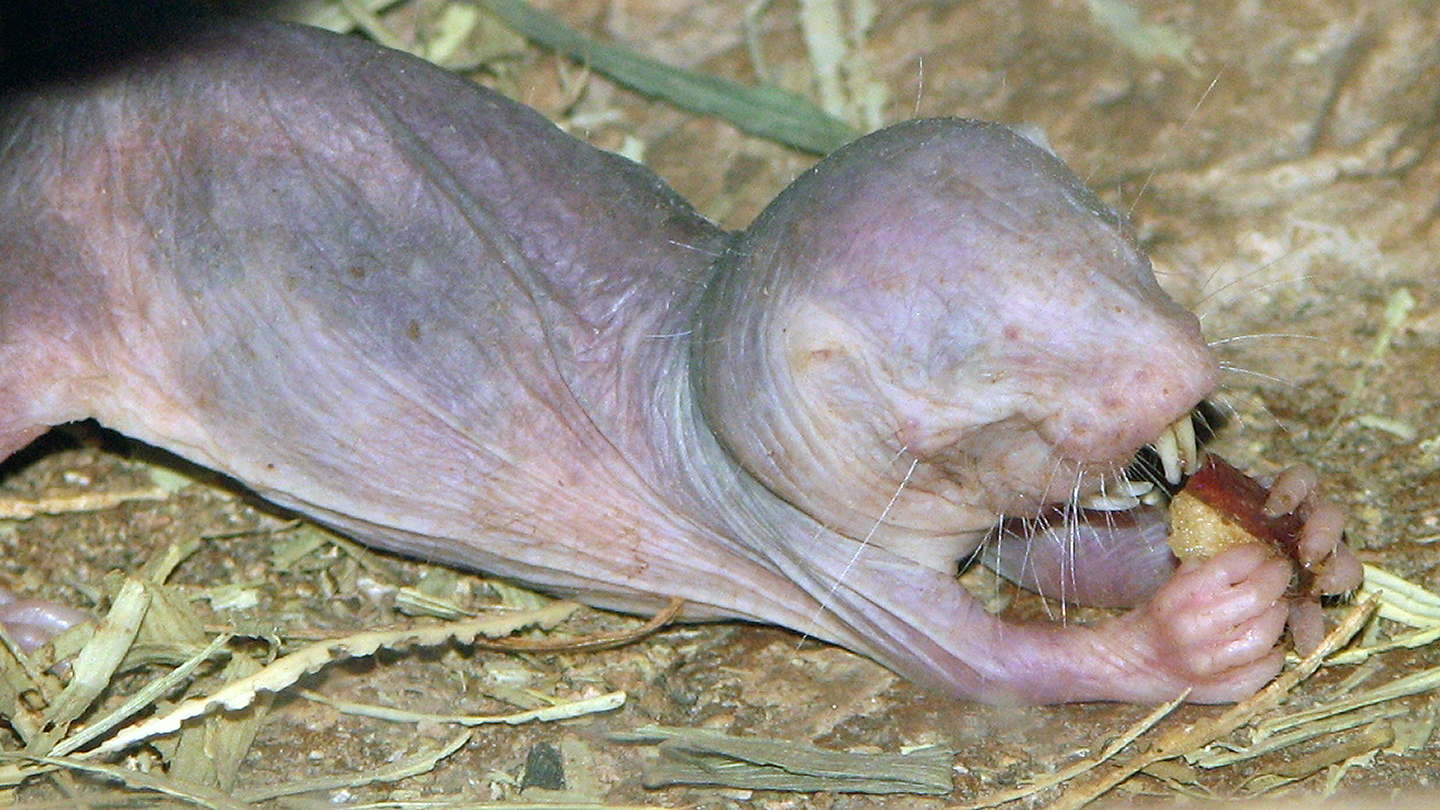The image depicts a highly underdeveloped, hairless rodent-like animal lying on a patch of brown dirt interspersed with sparse, pale grass. The animal's skin is mostly transparent and wrinkled, featuring a range of pink and dark purple hues, along with visible veins beneath the surface. Its eyes are not yet visible, giving the appearance of pure skin without any visual organs. The creature has developed long, human-like fingers at the ends of its arms, which it uses to hold a piece of fruit resembling an apple, with red skin and white flesh. The animal is in the act of bringing the fruit to its mouth. Prominently, it has two large fang-like teeth on the top and several matching teeth on the bottom, suggesting it is capable of biting into its food. No ears are visible, and there are no markings or signs to indicate the species of this unidentified, fetus-like animal.